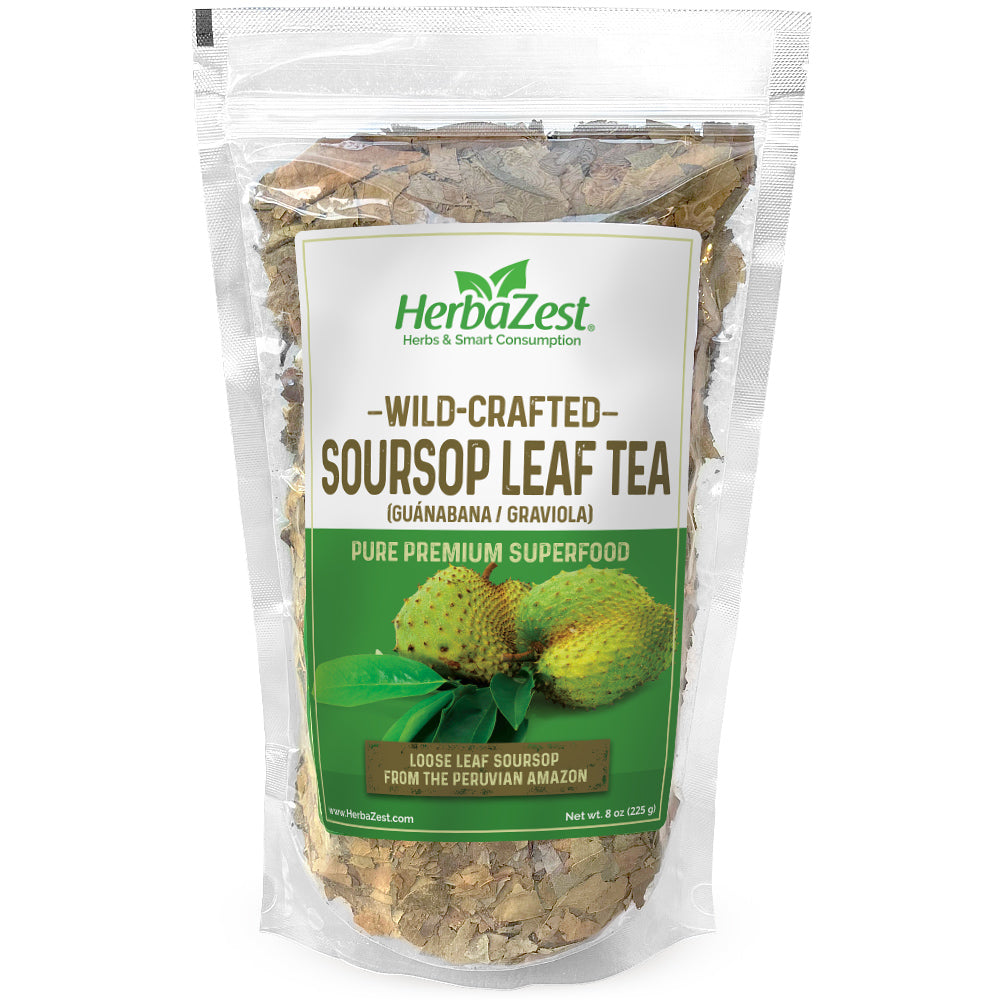The image depicts a stock photo of a resealable clear plastic bag containing brown and green dried leaves, labeled as Wild-Crafted Soursop Leaf Tea from Herba Zest under their Herbs and Smart Consumption line. The package, weighing 8 ounces (225 grams), features a split label: the top half with a white background displaying "Herba Zest Herbs and Smart Consumption" in green text and "Wild-Crafted Soursop Leaf Tea" in brown text, while the bottom half is green with the gold text stating "Pure Premium Superfood" and "Loose Leaf Soursop from the Peruvian Amazon." The label also includes an image of a soursop fruit—a spiky green fruit next to its leaves—highlighting its premium and superfood qualities. A ziplock seal secures the bag, allowing a clear view of the tea leaves inside.